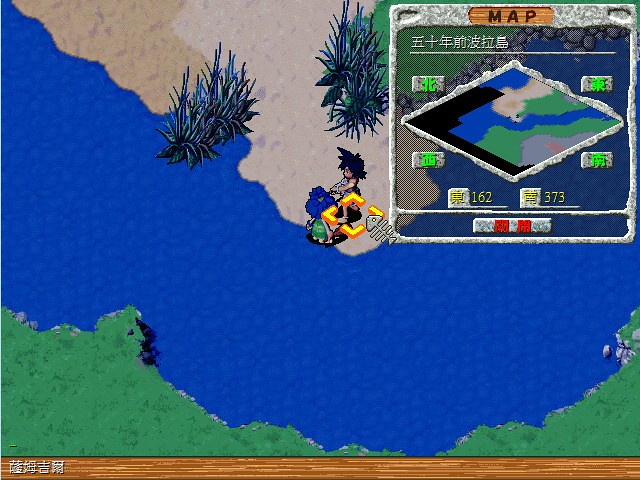The image appears to be a screenshot from a rudimentary, old-school computer or video game. Dominating the center, there is a character with black spiky hair, reminiscent of anime, who seems to be riding or standing on a machine. Opposite him stands another character with blue hair in a green dress. The background showcases a basic landscape with green land, a blue expanse of water, gray sand-like areas, and patches of oversized shrubs. An orange-yellow square with a fishbone symbol points towards the characters next to the water, suggesting they're near a beach with scattered bushes.

In the bottom left corner, there are white Chinese characters overlaid on a brown wood-like strip. Towards the top right, a secondary window displays a map labeled "Map" in English, featuring more Chinese characters and numbers "162 373." This map outlines the surrounding area with colors indicating different terrains: black, blue, green, white, and gray. The overall aesthetic and the interface evoke a nostalgic 1980s video game vibe.